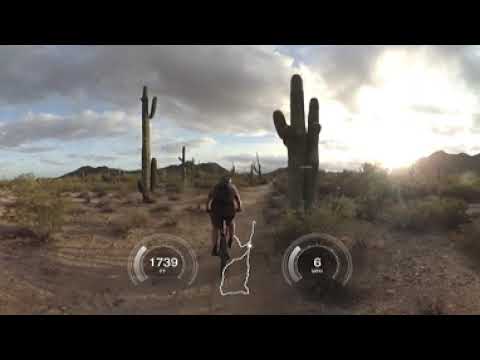The image captures a solitary bicyclist traversing a dirt trail through a desert terrain, characterized by sparse vegetation, including several large cacti and green bushes. The cyclist, seen from the back and clad in dark attire and shorts, carries a backpack as he pedals away from the viewer. The trail, faintly outlined in white, snakes directly through the arid landscape, flanked by cacti, with one prominent cactus on the middle right displaying a central tall stalk and three shorter arms. Above, the sky is a contrast of bright sunlight and dramatic clouds, transitioning from dark gray on the left to lighter white on the right. Rocky outcrops punctuate the terrain, with distant mountains visible in the far left corner. Adding a modern, digital touch to the natural scene, two translucent gauges overlay the image: one on the left displaying the number 1739, and another on the right showing the number 6 accompanied by unreadable text underneath.